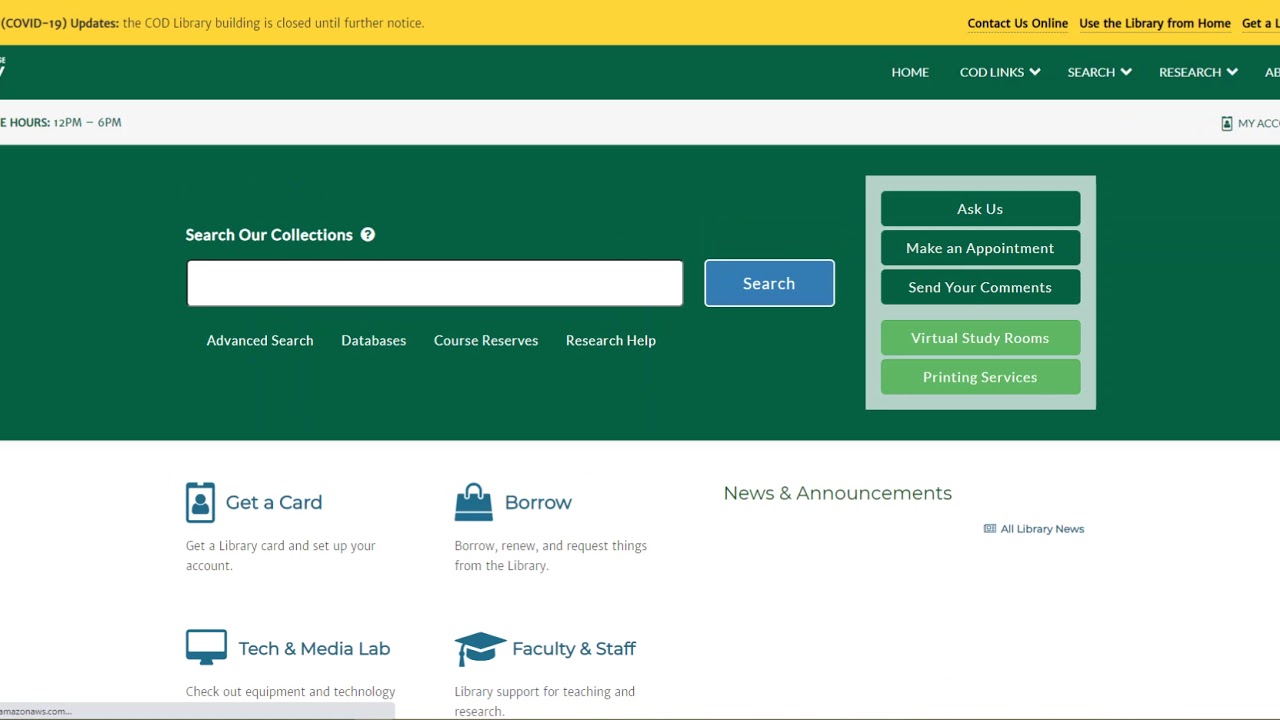A detailed screen capture of a website providing COVID-19 updates from the COD library is displayed. Dominating the top section of the screen is a bright yellow banner with the notice "The COD library building is closed until further notice" clearly written in bold black letters. 

Beneath this, another horizontal banner stretches across the screen in a forest green color. On the right-hand side of this banner, white text provides a menu with categories: Home, COD Links, Search, Research, and an additional label that is partially off-screen. 

Above the yellow banner, another line of text in black on yellow reads: "Contact us online, use the library from home, and get a," with the remainder of the message cut off and not visible. 

Directly below the green banner, a slim white banner contains important information. On the left, it states "Hours: 12 p.m. to 6 p.m.," while on the right, a "My Account" button is visible for user access.

Continuing the website theme, in the forest green section, a central white search bar prompts users with "Search Our Collection" written above it in white text. To the right of this search bar is a blue "Search" button. Additionally, options for "Advanced Search", "Database", "Course Reserves", and "Research Help" are listed below the search bar.

As the page continues downward towards the bottom, various icons and sections are available for navigation: "Get a Card," "Tech and Media Lab," "Borrow," "Faculty and Staff," "News and Announcements," and a "Next" button for further exploration.